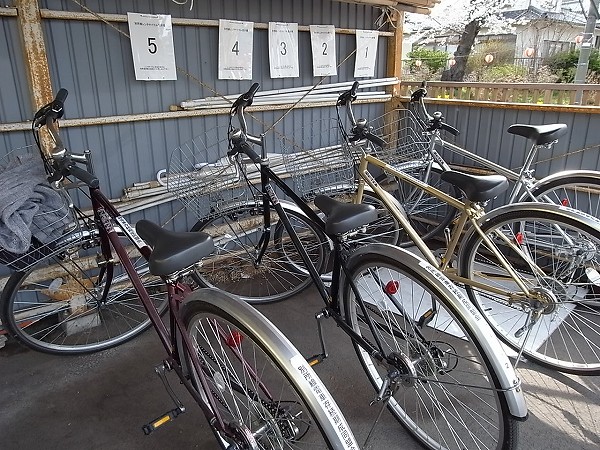The image depicts a landscape-oriented, daytime photograph of four bicycles parked in a designated area, which appears to be either a garage or a shed with blue-gray siding. Above the bicycles, there are laminated white sheets of paper displaying the numbers one through five, in descending order from right to left. Each bike has a wire basket and a bell attached to the front, and their kickstands are all down, indicating they are stationary. The bicycles, which are lined up side by side, feature differently colored frames—burgundy, black, gold, and silver. The far-left bike has a towel placed in its basket. The scene might suggest a bike rental facility, potentially situated in a neighborhood setting, intended to highlight the available bikes for sightseeing or local transportation. Additionally, white shelving with poles is visible, adding to the organized layout of the area.